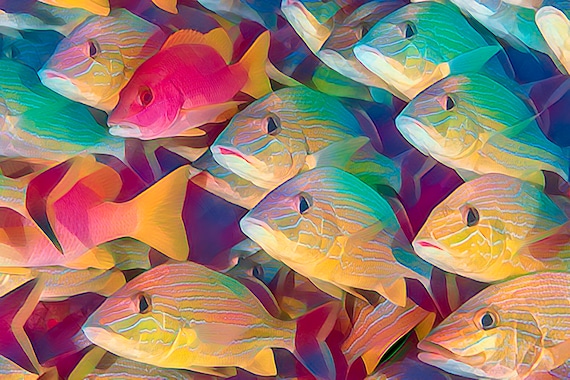The image portrays a meticulously crafted piece of artwork, likely a 3D rendering or a watercolor painting, showcasing a vivid school of fish that bear a strong resemblance to goldfish or koi. There is a wide spectrum of colors depicted in the fish, ranging from shades of turquoise blue at the tops, transitioning into purples, yellows, and bright sun-like yellows. The fish are all swimming closely together from right to left, creating a dynamic and cohesive movement across the frame. Their eyes are predominantly dark green or black, with each fish showing only one eye visible. The hues of the fish blend seamlessly into one another, with greens melding into bright yellows and purples fading into greens. The overall composition is vibrant and fluid, leaving the impression of a shoal of diverse, yet harmoniously colored fish.